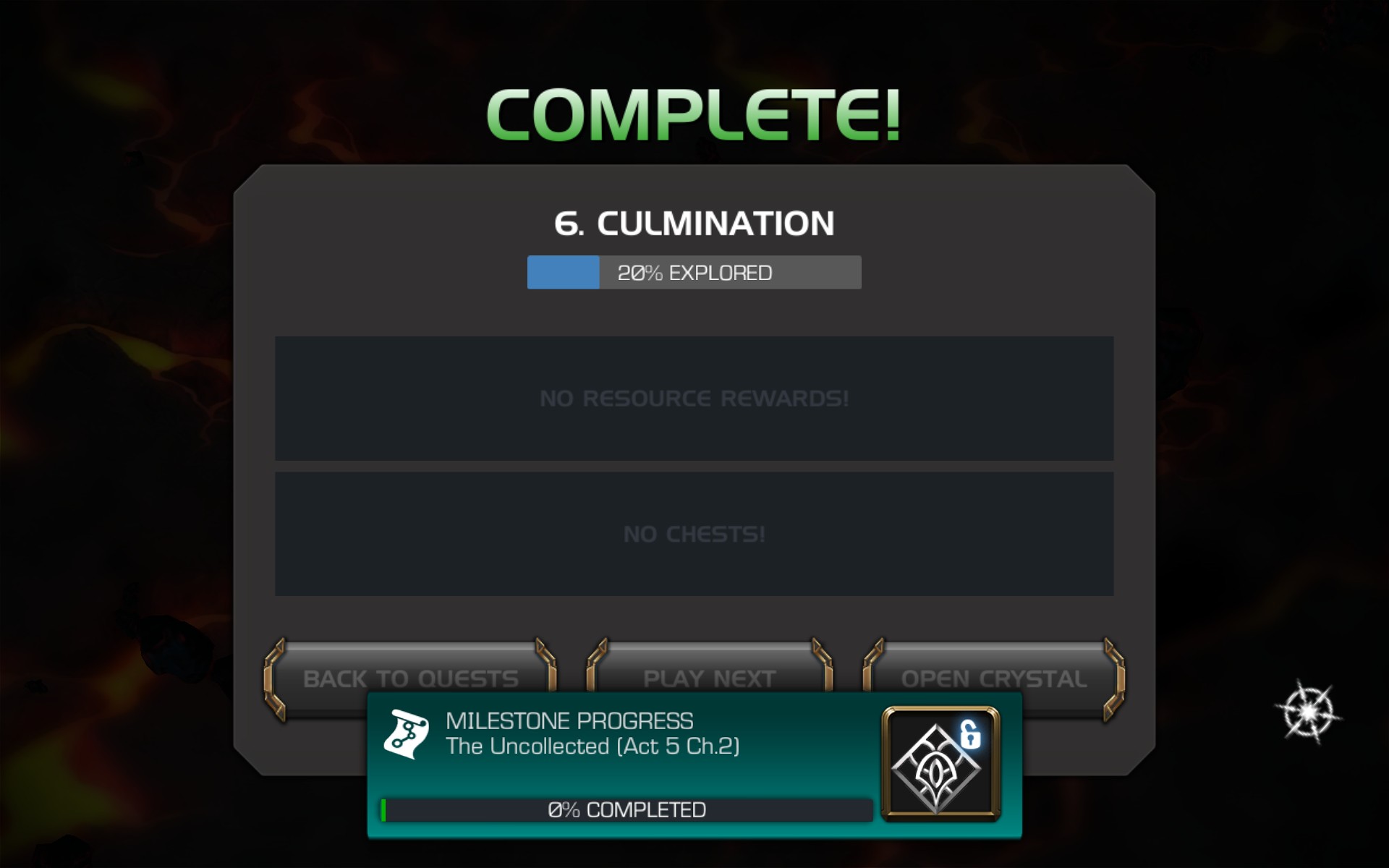This image is a screenshot from a video game interface featuring a blackish background and bright lime green text. At the top center, "Complete!" is prominently displayed. Just below that, within a green frame, it reads "Six Dot Accumulation." A progress bar beneath this frame shows "20% Explored," where the bar is predominantly gray with a 20% blue fill. Below the progress bar, there are two grayed-out sections that state "No Resource Rewards" and "No Chests." Further down, three smaller buttons with rounded edges and gold borders are aligned. The buttons read: "Back to Quests" on the left, "Play Next" in the center, and "Open Crystal" on the right. To the right side of the screen, there's a silver star encircled, and near the bottom middle, a greenish box displays "Milestone Progress: The Uncollected (Act 5, Chapter 2)" with "0% Completed" written in white letters on a gray bar. To the right of this gray bar, there's a gold square with a white unlock icon and a silver diamond emblem featuring a blue unlock symbol.